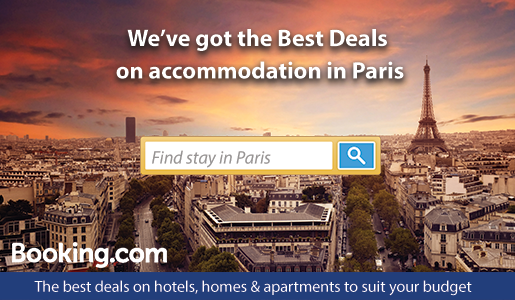A vibrant, detailed advertisement for booking.com is depicted against the mesmerizing background of Paris, France. The foreground features prominent white text proclaiming, "We've got the best deals on accommodation in Paris," bordered by alternating white and yellow edges. Below, in a blue square lined with white, the text urges viewers to "Find Stay in Paris." On the bottom left, the booking.com logo is clearly visible. 

An additional blue-bordered message at the bottom of the image invites viewers to explore "the best deals on hotels, homes, and apartments to suit your budget." The backdrop offers a stunning view of Paris, with the iconic Eiffel Tower visible to the right, set against a dramatic purple and blue sky, punctuated by red-tinted clouds. The cityscape features densely packed urban buildings, streets bustling with activity, and green trees adding touches of nature. The buildings showcase white walls, black rooftops, and numerous windows. The roads are filled with vehicles, and the urban sprawl seems to stretch endlessly under the evening sky.